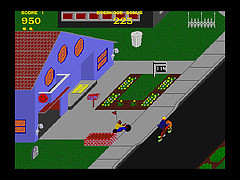This image presents a detailed scene reminiscent of an old-school arcade video game, framed by a black border on all four sides, encapsulating a square format. The primary focus is a horizontally oriented environment with various elements interspersed throughout.

On the right, a brown strip of earth can be seen, dotted with green hedges. Adjacent to this, a black road runs vertically with a cyclist riding along it. Moving further left, a light gray sidewalk is depicted, paralleled by another cyclist in a yellow shirt navigating his way along a path bordered by a patch of garden. This garden features a well-defined contrast of brown soil and green foliage.

Adjacent to the garden, there is a blue house with distinctive features including a brown roof, orange circular and rectangular windows, and set against a backdrop of a lush green field. Positioned above the house, the scene transitions into open grassy terrain.

Overlaying the landscape, the left-hand side of the image prominently displays the text "Score 950" in bold yellow font, while the center of the image features the number "225," also in yellow. These textual elements evoke the scoring systems typically found in classic arcade games, adding an additional layer of nostalgia to the scene.